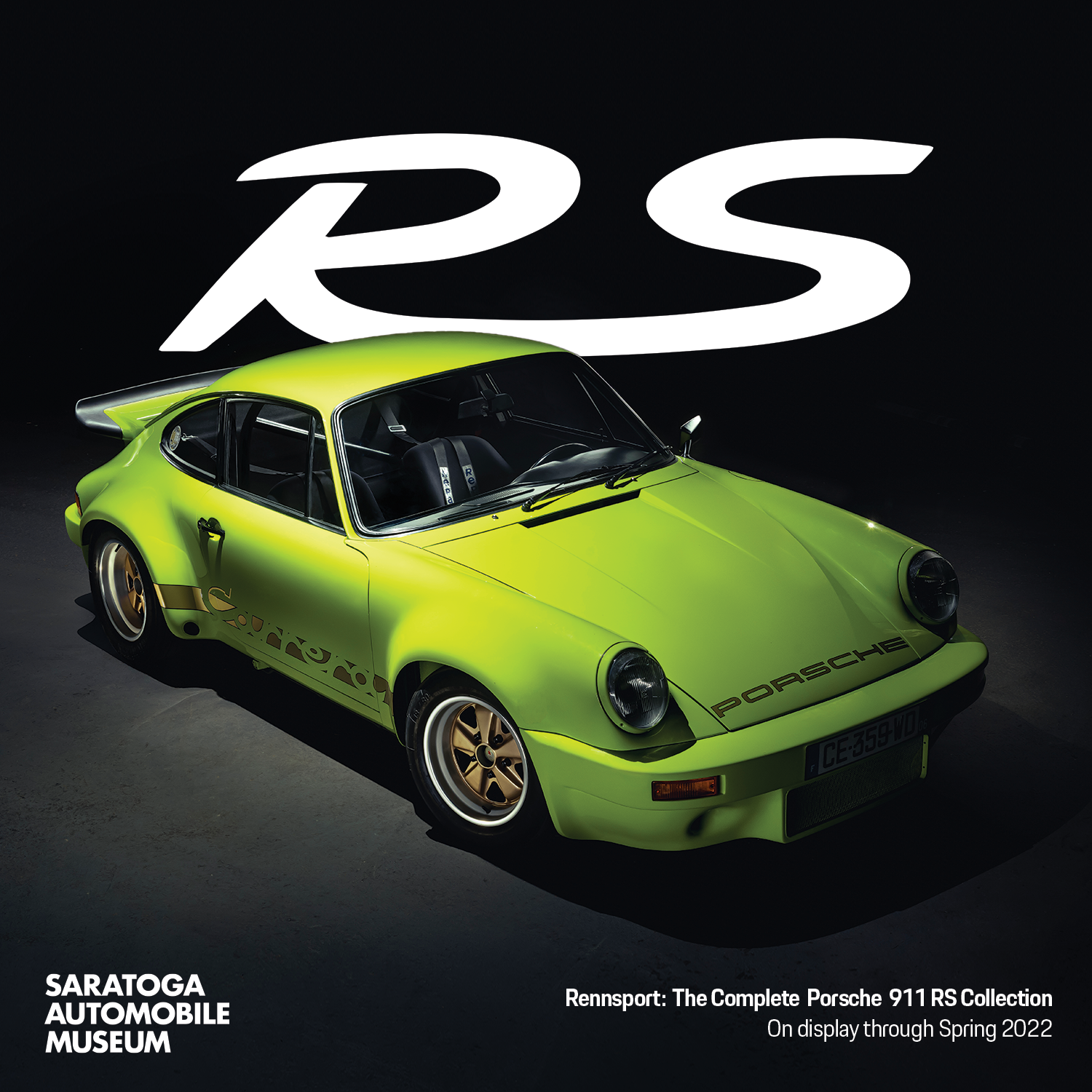This image from the Saratoga Automobile Museum showcases the prestigious Rennsport exhibit, featuring the complete Porsche 911 RS collection on display for Spring 2022. Central to the photo is a striking lime green Porsche Carrera, distinguished by its black interior and elaborate gold detailing on the tires, door handles, and the Porsche Carrera insignia. The car features a pronounced rear spoiler and gold-centered wheels with silver rims. A prominent 'RS' in white cursive adorns the top of the image above the car, adding a touch of elegance. Below this, the license plate reads CE359WO. The overall presentation is designed to highlight the sleek, high-performance nature of these iconic cars, promising to draw considerable attention from visitors.